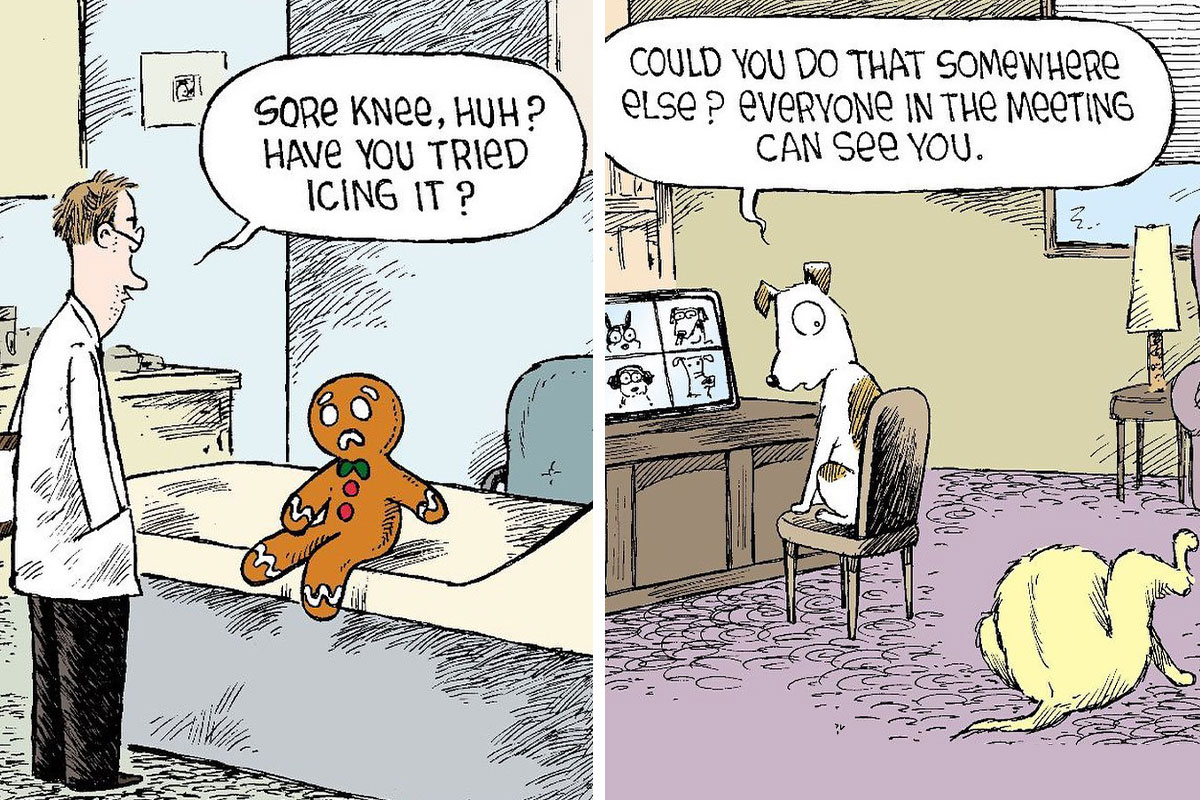In a two-panel newspaper comic strip, the left panel features a scene in a doctor's office, with the central focus on a gingerbread man cookie sitting on the examination table. The doctor, depicted with a scruffy face, brown hair, glasses, and dressed in a white lab coat and black pants, is looking at the gingerbread man and humorously says, "Sore knee, huh? Have you tried icing it?" The gingerbread man, adorned with white icing, red buttons, and a green bow tie, appears to be the only element in color against the blue-beige office backdrop. The right panel showcases a home setting with a dog sitting in a chair in front of a computer that displays a Zoom meeting featuring four dogs. The main dog, which is white with brown spots, is looking backwards at another yellow dog on the floor, who is licking itself. The exasperated dog at the computer says, "Could you do that somewhere else? Everyone in the meeting can see you." The home setting includes a purple carpet and a yellow wall, adding vibrant details to the scene.